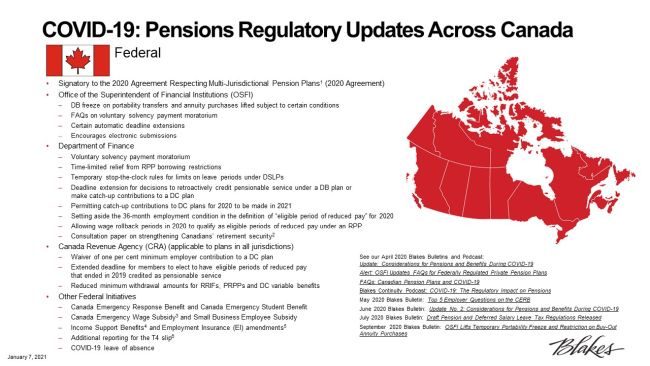This image features a detailed list titled "COVID-19 Pensions Regulatory Updates Across Canada" prominently displayed. At the top of the document, a Canadian flag accompanies the title "Federal." To the upper right section of the image, there is a map of Canada shaded entirely in red.

The main content of the document begins with a section labeled "Signatory to the 2020 Agreement Respecting Multi-Jurisdictional Pension Plans" and mentions the "2020 Agreement" managed by the "Office of the Superintendent of Financial Institutions." Below this heading, there are several detailed points, including:
- A note about the DB freeze on portability transfers and annuity purchases being lifted under certain conditions.
- FAQs addressing the voluntary solvency payment moratorium.
- Details on certain automatic deadline extensions and encouragement of electronic submissions.

Following these points, the document shifts focus to updates from the "Department of Finance," which include:
- Information on the voluntary solvency payment moratorium.
- Time-limited relief from Registered Pension Plan (RPP) borrowing restrictions.
- Temporary "stop-the-clock" rules regarding limits on leave periods under Deferred Salary Leave Plans (DSLPs).

The content proceeds in a similar comprehensive manner down the rest of the page, detailing regulations and updates stemming from the impact of COVID-19 on pension plans in Canada.